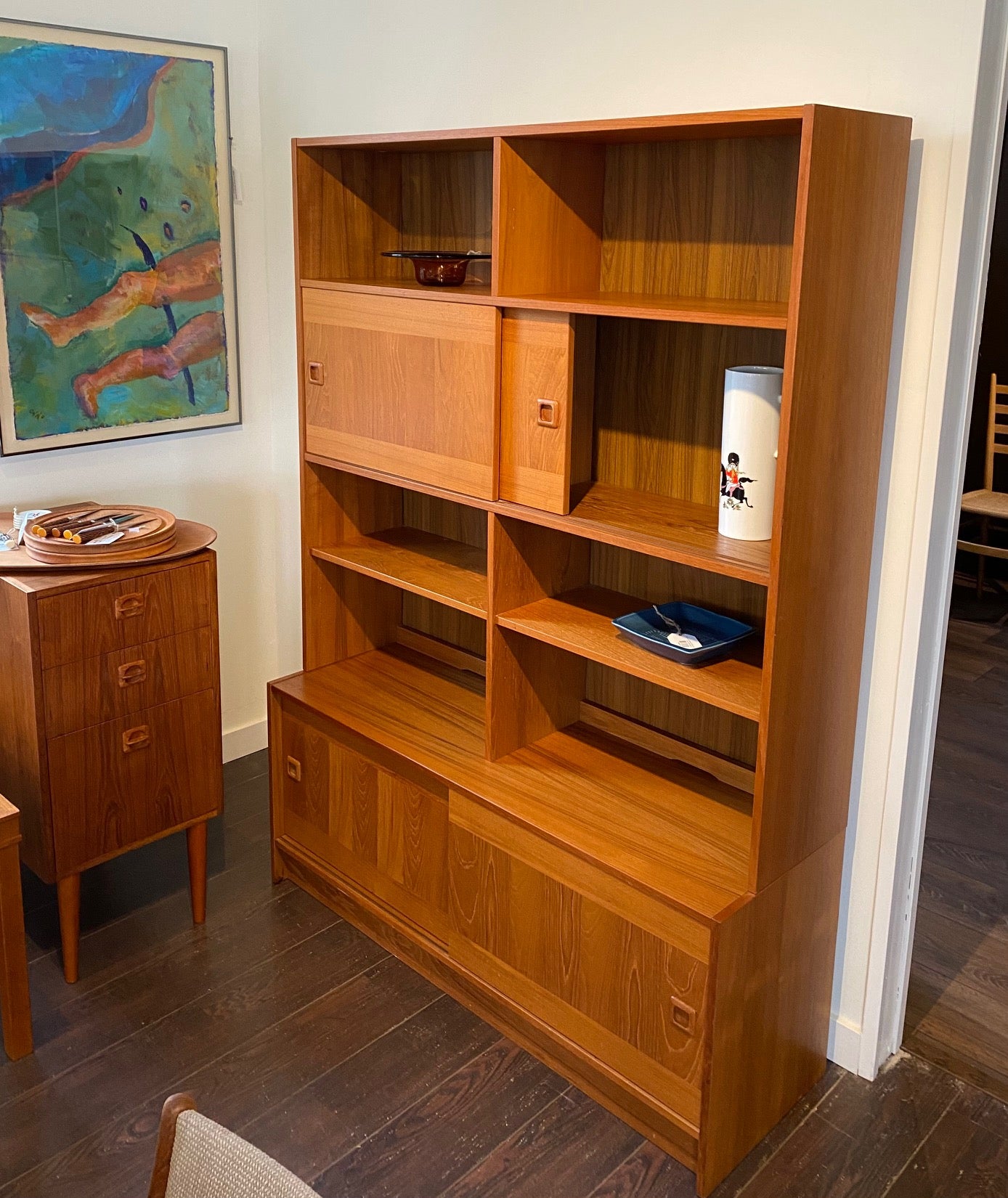This color photograph, in portrait orientation, captures a detailed view of a room, likely an office or bedroom, featuring a large teak wood bookcase against the back wall. The bookcase is characterized by multiple shelves, some of which are open, while others are enclosed with sliding doors that are light wood in color. On the rightmost shelf, there's a notable white cylindrical item, and on the leftmost top shelf, a small dark glass vase is visible. Beneath these, the second level down on the right side holds a blue rectangular piece of ceramic dishware, and there’s another round circular object near it. 

The floor is comprised of dark wood planks, grounding the space with a warm, earthy tone. Adjacent to the bookcase on the left side, the image includes a matching side table with three pull-out drawers and pointed legs, atop which sits a tray. Above this side table, there is a detailed piece of artwork, incorporating shades of brown, blue, and green, depicting an abstract view of a man's legs next to a pool. This artistic element adds a pop of color and a touch of modern representational realism to the room's decor.